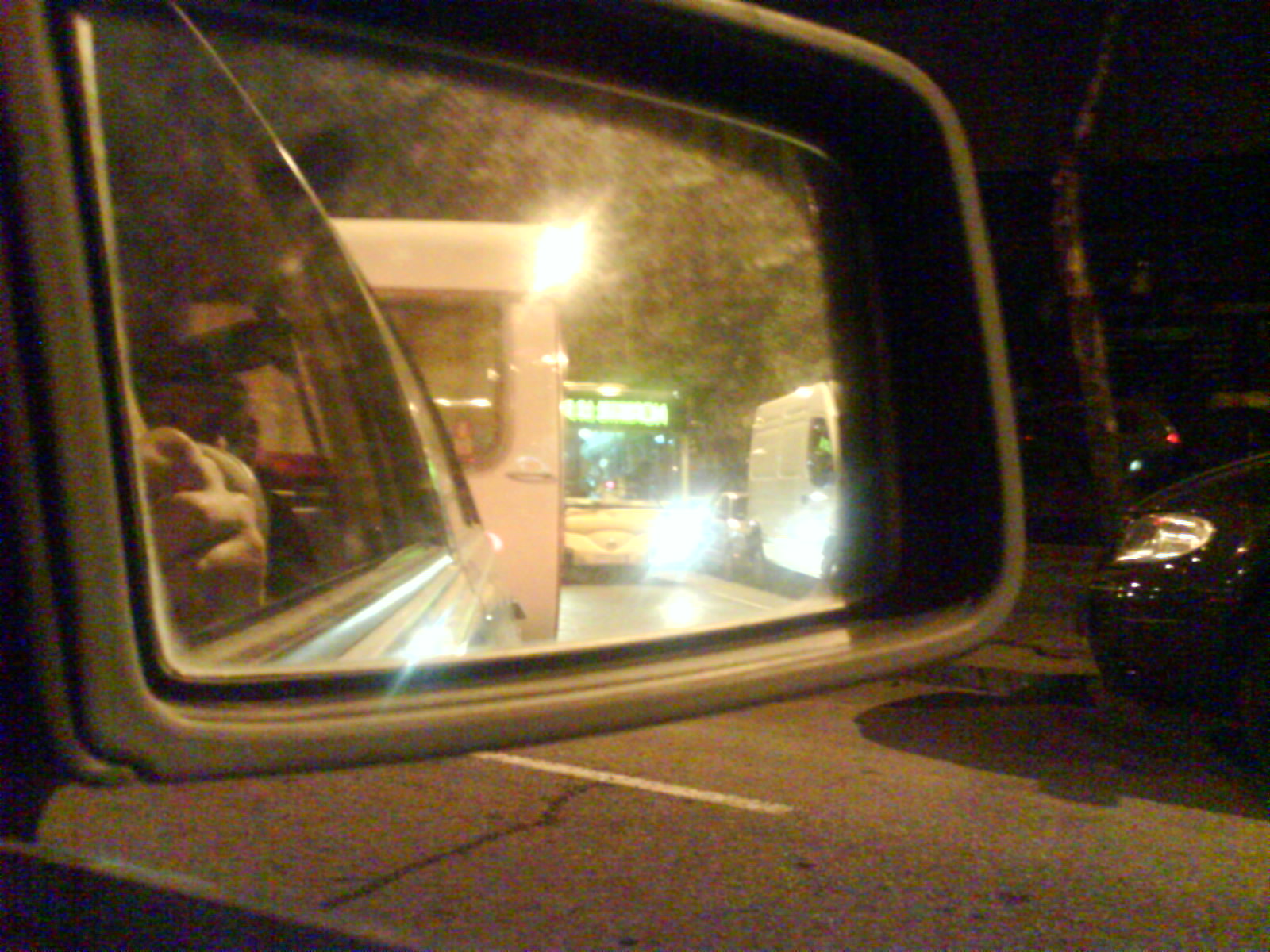A close-up view captures the reflective surface of a rearview mirror, showcasing a bustling urban scene. In the mirror's reflection, a large city bus, with its headlights and interior lights on, navigates through a narrow, two-lane street lined with cars parked along both curbs. The bus's digital display is prominently visible across the top. Alongside the curb on the right, the front end of a parked car is seen, with a man's face visible behind the wheel. Behind this car, another vehicle is towing a white, rounded RV, or possibly an unusually shaped bus, adding to the complexity of the scene. A woman's face appears in the bottom right corner of the bus's windshield, adding a human element to the reflective image.